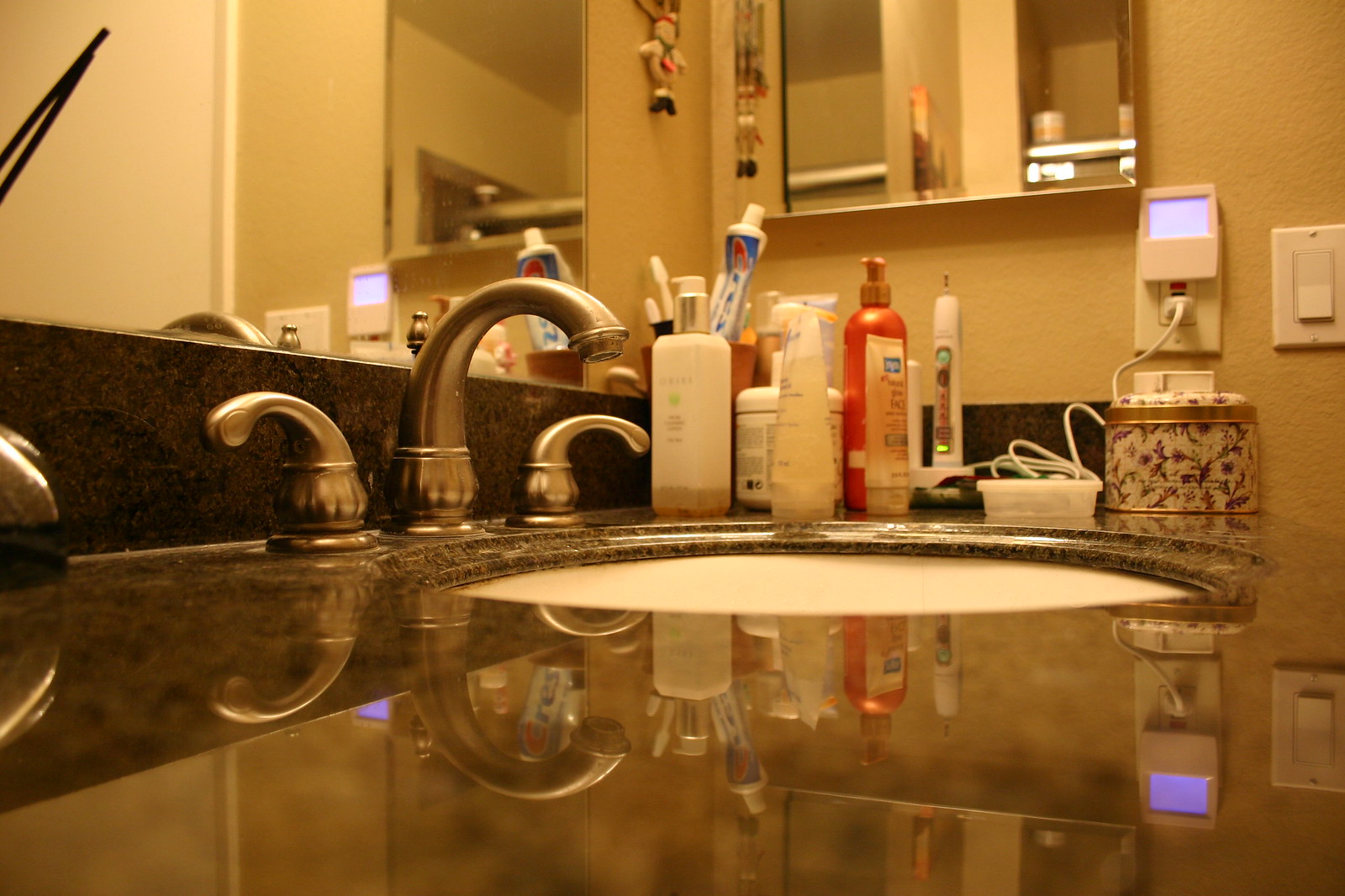This angled eye-level photograph captures a detailed view of a bathroom sink from the left corner, spanning towards the back right corner. The countertop and backsplash of the sink are made of luxurious brown granite. A tall, rounded silver faucet with intricately designed bases anchors the scene, accompanied by matching rounded silver handles.

At the top left of the image, a portion of a large bathroom mirror is visible, reflecting light and adding depth to the space. Centrally, on another wall, the bottom part of a glass medicine cabinet appears, situated above hanging jewelry, including a visible necklace against the tan wall. To the left of this necklace, a small snowman decoration dangles from an unseen fixture, adding a whimsical touch.

The bottom center of the photograph showcases a variety of personal products cluttering the upper right corner of the sink. Among these items are a nearly empty tube of Crest toothpaste stored vertically in a cup, two white toothbrushes facing the wall, several white and orange bottles, and a small white container with a screw cap. Additionally, a plug is inserted into an outlet on the left side, with a white square nightlight emitting a blue LED glow above it.

Towards the right corner, a rounded gold metal canister with a floral motif on an ivory background sits on the countertop, its contents obscured from view. Adjacent to it is a small plastic Tupperware container. The far right corner reveals a push-button outlet with a rectangular front, designed for ease of use without the need for flipping switches.